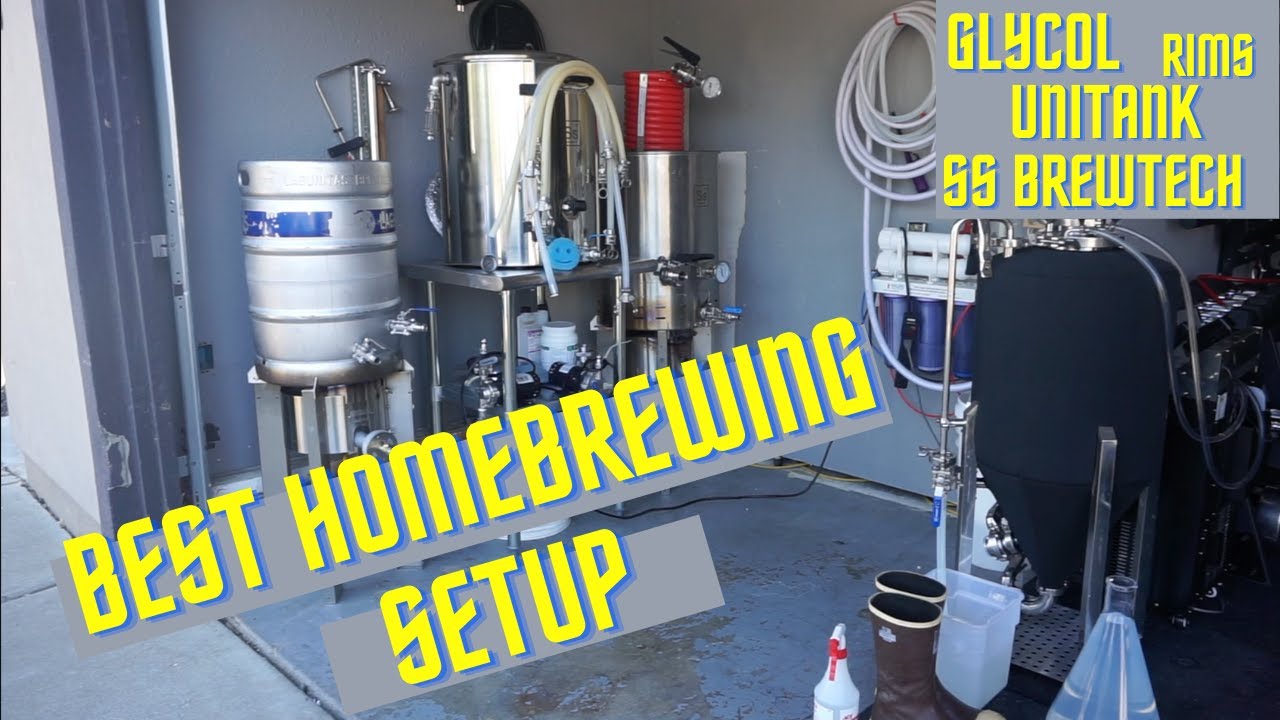The image titled "Best Home Brewing Setup" prominently features large yellow lettering on the left side and the text "Glycol Rims Unitank SS Brewtech" in the upper right corner, indicating it is an advertisement for high-tech home brewing equipment for beer. The scene is a highly detailed, stainless steel brewing setup that appears meticulously clean and advanced. It includes kegs, brewing vats, and distilling equipment, with computerized controls and filtration systems visible on the right side of the image. The floor resembles concrete, perhaps suggesting a garage setting, and it's dotted with practical items including a pair of rubber work boots, a spray sanitizer bottle, and a red hose on a metal shelf. Additionally, there are black-clothed tanks, tubes hanging against a gray wall, and various scientific instruments such as beakers and pressure gauges, emphasizing the precise and technical nature of this home brewing setup.